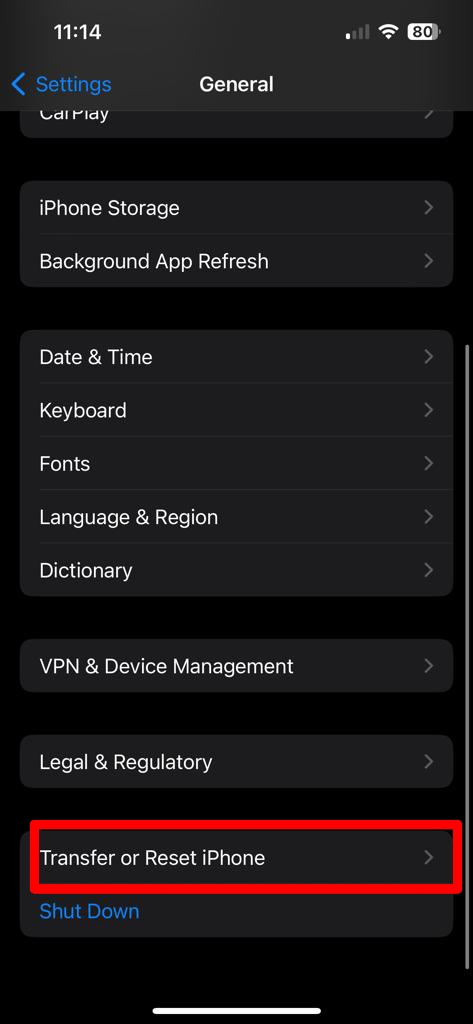This detailed screenshot, captured at 11:14, showcases an iPhone with an 80% battery and a full signal. The screen is set within the "Settings" app under the "General" section, displaying various menu options against a black-brown background. At the top, "iPhone Storage" is listed with an arrow indicating further access. Below it, "Background App Refresh" is similarly indicated with an arrow. Following these, the menu lists "Date & Time," "Keyboard," "Fonts," "Language & Region," and "Dictionary," each accompanied by an arrow for additional configuration. Near the end of the list, the "VPN & Device Management" and "Legal & Regulatory" sections also feature navigational arrows. Highlighted prominently in red, the "Transfer or Reset iPhone" option appears just above the “Shutdown” button. This highlighted section is the focal point, suggesting it is the desired selection for the user.